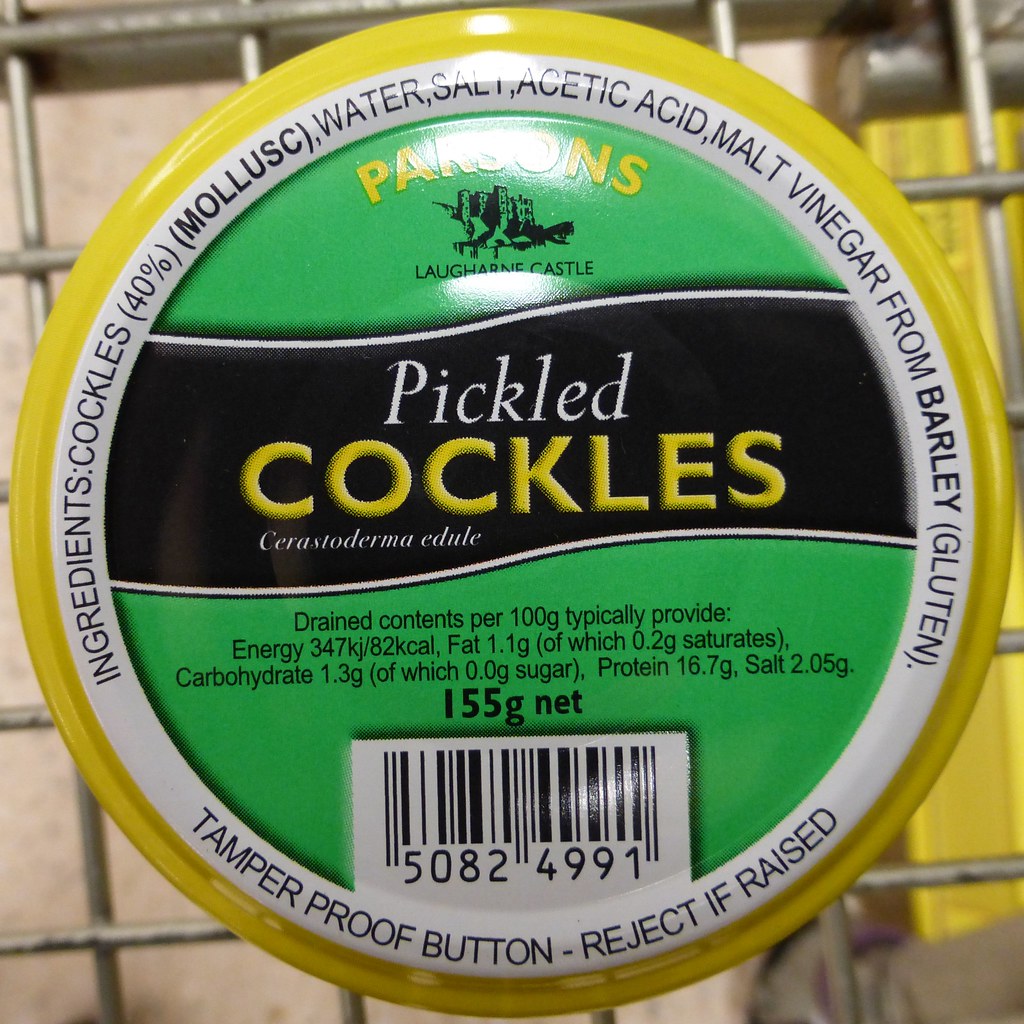The image depicts a jar of pickled cockles from the brand Paxsons. The jar is round with a yellow lid and a white inner circle on top that is labeled. The lid prominently features the product name, "Pickled Cockles," and below it, the scientific name "Cerastoderma edule." The jar sits on a mesh wire shelf, providing a textured background. 

Around the lid, the ingredients are listed: "Cockles (40%) (mollusk), water, salt, acetic acid, malt vinegar from barley (gluten)." Additional nutritional information is provided: "Drained contents per 100 grams typically provide: Energy 347 kJ / 82 kcal, fat 1.1 g (of which 0.2 g saturates), carbohydrate 1.3 g (of which 0.0 g sugars), protein 16.7 g, salt 2.05 g." 

At the bottom of the white circle, it states, "Tamper-proof button – reject if raised." The net weight of the jar is indicated as "155 g," and a UPC barcode with the numbers "5082-4991" is also present. A partially visible picture of a UK castle can be seen in the background, adding a regional touch to this specialty food item.